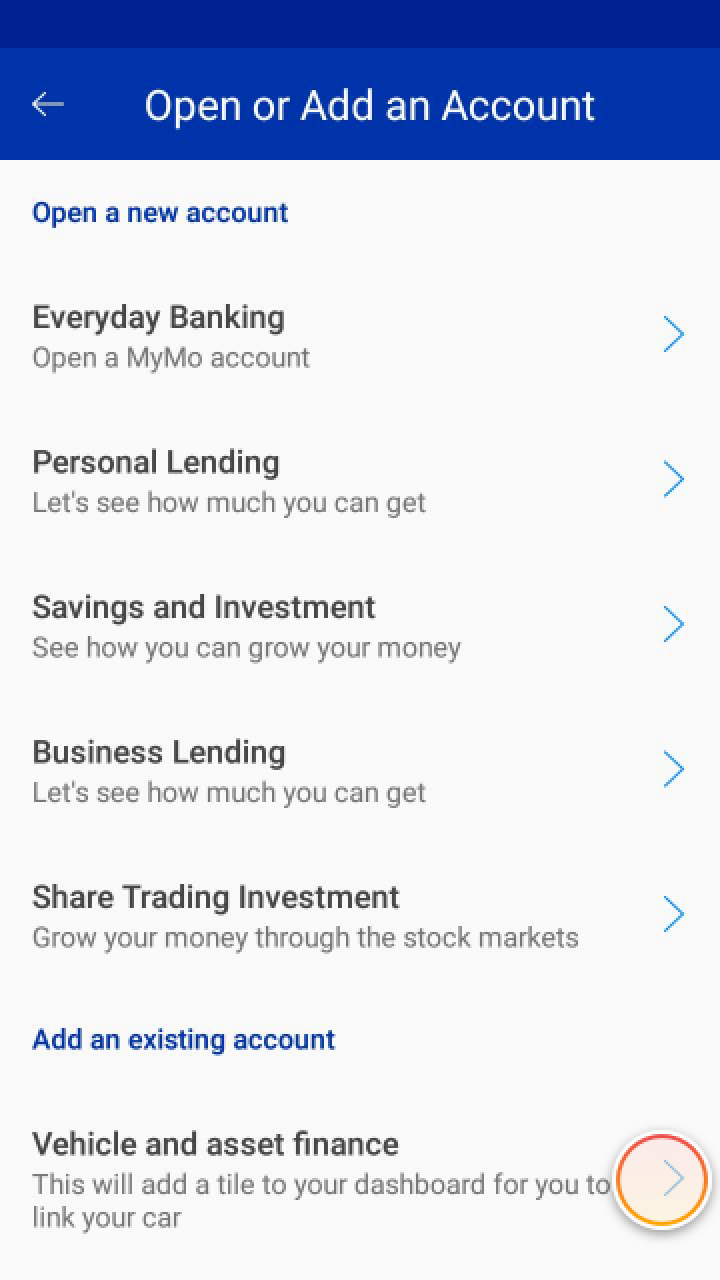Screenshot of a mobile app interface featuring various financial service options on a blue banner at the top with the text "Open or add an account" and a white arrow pointing left. In the center of the banner, the option "Open a new account" is prominently displayed.

Below the banner, several options are presented:

1. **Everyday Banking:**
   - "Open a MyMo account" with a blue arrow to the right.

2. **Personal Lending:**
   - "Let's see how much you can get" with a blue arrow to the right.

3. **Savings and Investment:**
   - "See how you can grow your money" with a blue arrow to the right.

4. **Business Lending:**
   - "Let's see how much you can get" with a blue arrow to the right.

5. **Share Trading Investment:**
   - "Grow your money through the stock markets" with a blue arrow to the right.

6. **Add an Existing Account:**
   - Text in blue letters positioned centrally on the screen.

7. **Vehicle and Asset Finance:**
   - Description: "This will add a tile to your dashboard for you to link your car."

At the bottom of the screen, there is a circular button featuring a gradient from white to faded orange, possibly intended for additional functionality not specified in the image description.